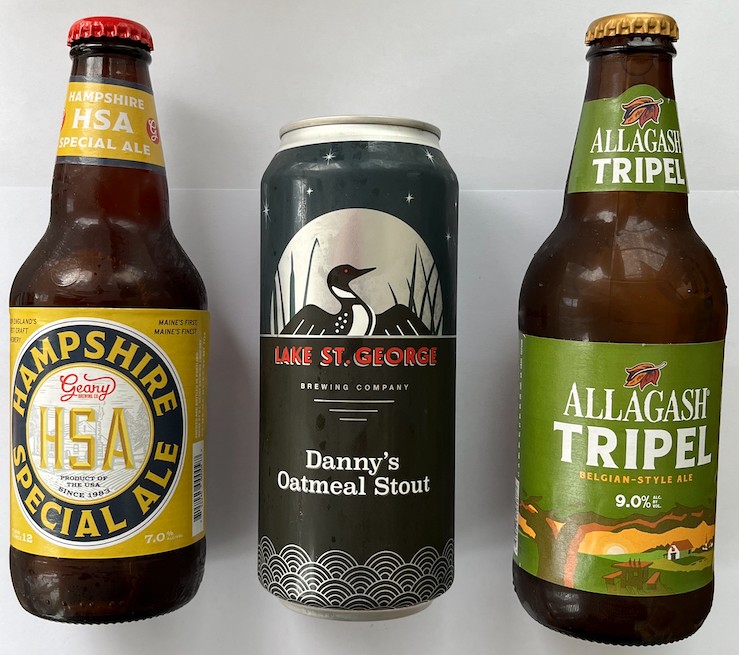The photograph showcases three distinct, cold and sweating beers, side by side with a small gap between each. On the left, there's a brown glass bottle featuring a mustard, white, and blue label, with "Hampshire Special Ale" encircling a black circle highlighted by gold text and "HSA" in the center. The middle item is a sleek black aluminum can labeled "Lake St. George Brewing Company, Danny's Oatmeal Stout," adorned with a red and white logo depicting a silhouette of a goose or duck against a full moon, standing amidst tall reeds. On the right, there's another brown glass bottle with an olive green label, intricately designed with a scene of a cabin and picnic table beneath a tree with a setting sun, stating "Allagash Trippel Belgian Style Ale, 9%."